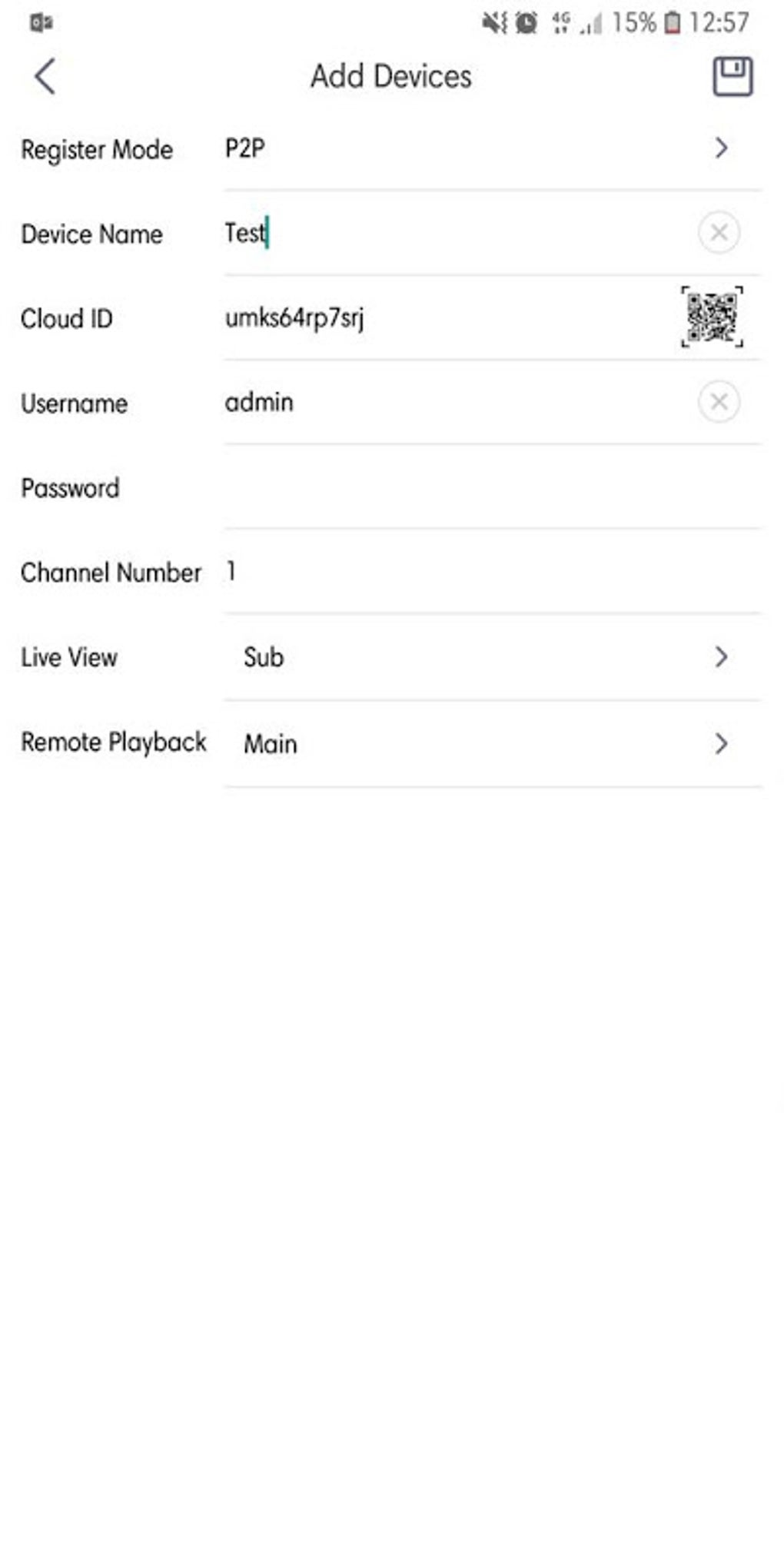The image displayed on either a phone or computer screen shows detailed system information. 

At the very top, a row of small icons is visible. Starting from the left, there are two small squares whose function is unknown. Moving right, the icons include a mute button, a Bluetooth indicator, a time display, a 4G signal strength indicator, and a battery icon showing 15% remaining, with the corresponding battery graphic nearly empty. The time indicated is 12:57.

Centered below these icons is the text "Add Devices." Below this heading is a detailed list of device configuration options. The first entry is "Register Mode," set to "P2P." Below this is "Device Name," currently entered as "Test," featuring an 'X' button to delete the entry. The next field, "Cloud ID," shows the ID "UMKS64RP7SRJ," with an option to expand to full screen on the right.

Following this, the "User Name" is listed as "admin," and the "Password" field is empty. The "Channel Number" is set to "1." Below this, "Live View" is set to "Sub," with a caret icon on the right for navigation. Finally, "Remote Playback" is configured as "Main," also accompanied by a caret icon for further actions.